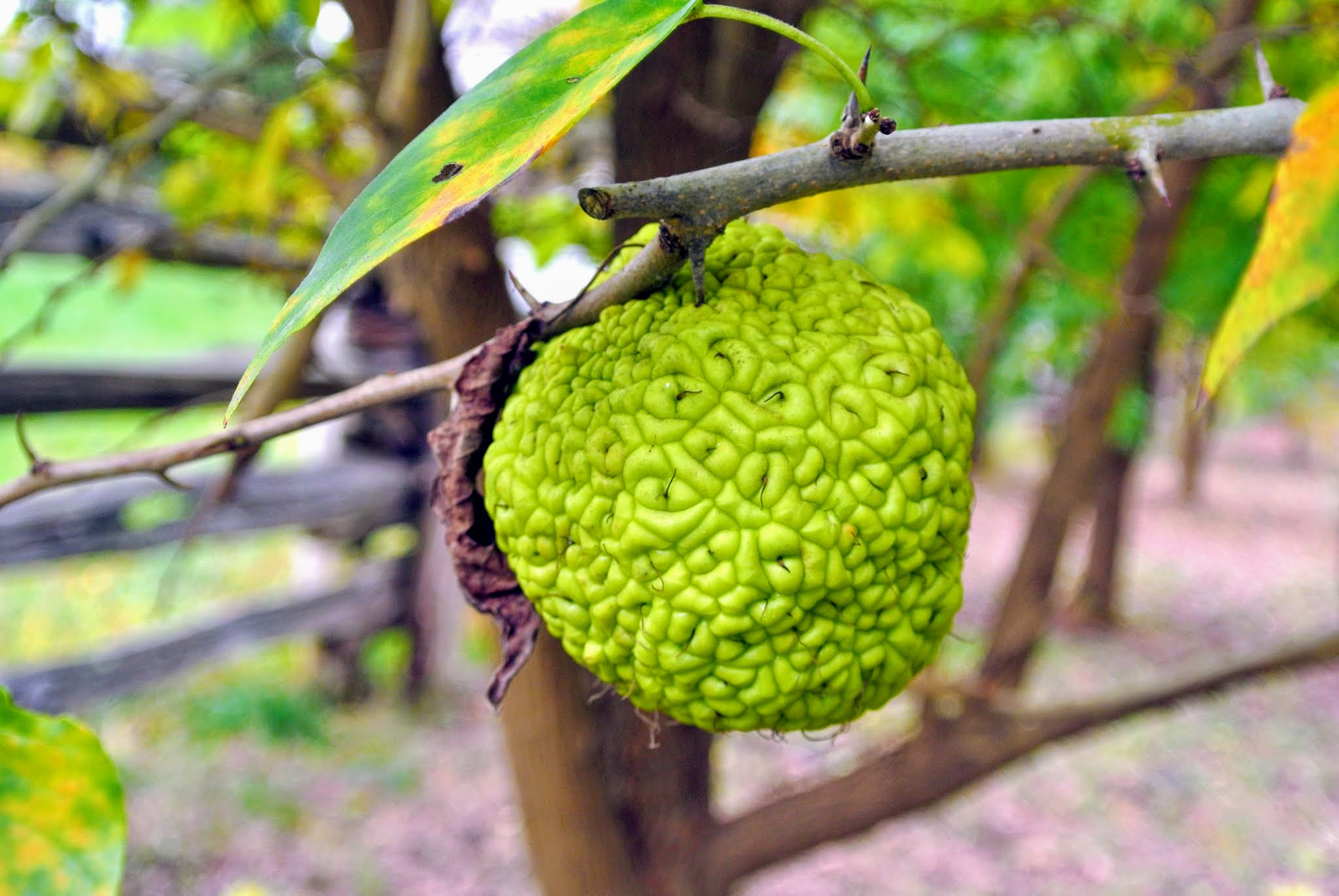In the image, we see a solitary, large, and green fruit hanging from a tree branch that appears somewhat mushed and wrinkled, resembling an oversized, segmented green apple or a breadfruit with a unique, squishy texture. The branch is gray, and other branches with leaves of varying colors—green, yellow, and orange—are intricately scattered throughout. A dried brown leaf is hanging beside the fruit, while a single green leaf can be seen above it. In the background, a dark wooden fence stands against a backdrop of a green environment, and the ground, partly gravel or light-colored dirt, has hints of red and green, suggesting fallen leaves or flowers. The overall atmosphere is clean and focused on the atypical appearance of the fruit.